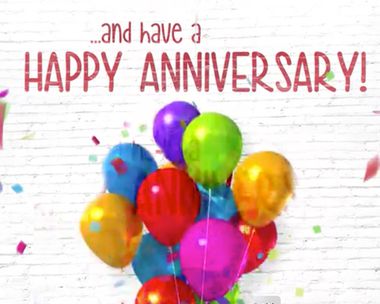The image is a color illustration with a white background featuring light gray, somewhat random horizontal lines that may appear as words but are largely unreadable and blurred. Centered prominently at the top in lowercase and dark reddish-brown ink are the words "dot dot dot and" followed by "HABE A." Below this text, in a much larger, all caps font, it declares "HAPPY ANNIVERSARY" with an exclamation point in the same reddish-brown color. Scattered throughout the scene is vibrant confetti in colors such as blue, green, red, yellow, and purple. The focal point in the bottom center is a cluster of colorful balloons, including red, gold, green, dark and light purple, aqua, and blue, all tied with strings. The balloons appear inflated and festive, enhancing the celebratory feel of the illustration. The entire image is presented in landscape orientation.